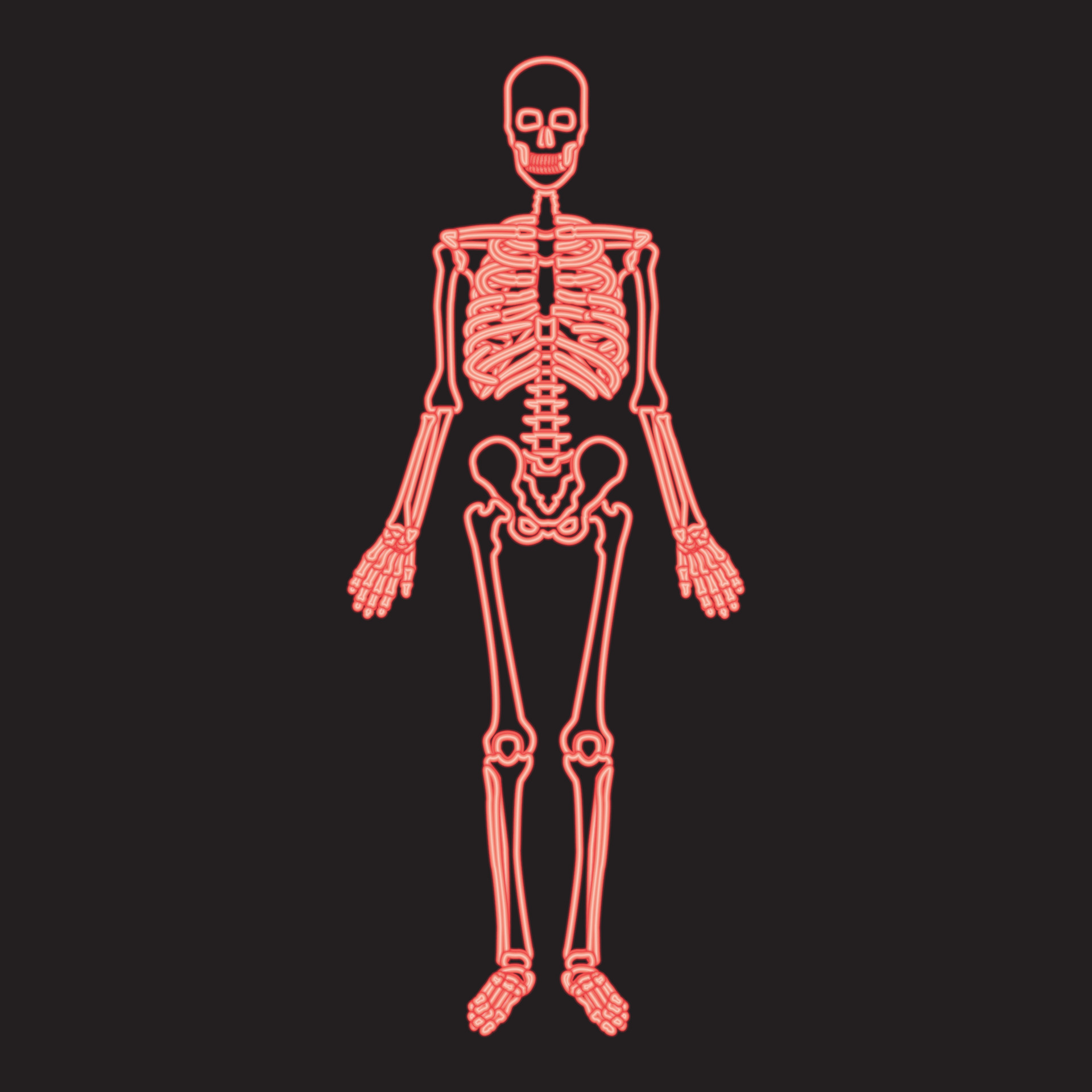The image depicts a highly detailed, brightly colored illustration of a human skeleton set against a stark black background. The skeleton, which is standing upright, is illustrated with neon-like lines that give it a glowing appearance. The bones, covered with a mixture of white and reddish-pink hues, are outlined in a bright hot pink, creating a vivid and striking contrast with the black backdrop. This effect emphasizes the intricate details of the skeleton, from the skull, jaw, and teeth to the clavicles, ribcage, and shoulder bones. The arms, shown descending to the forearms and hands, reveal detailed depictions of the various bones, particularly noticeable in the hands. The hip bones transition down to the femurs, knees, and eventually the foot bones, all rendered with a similar stylistic glow. While the illustration might evoke the feel of a medical teaching tool, its neon aesthetic and minimalist design—highlighting only the bone outlines—suggest a more artistic, LED-like representation.